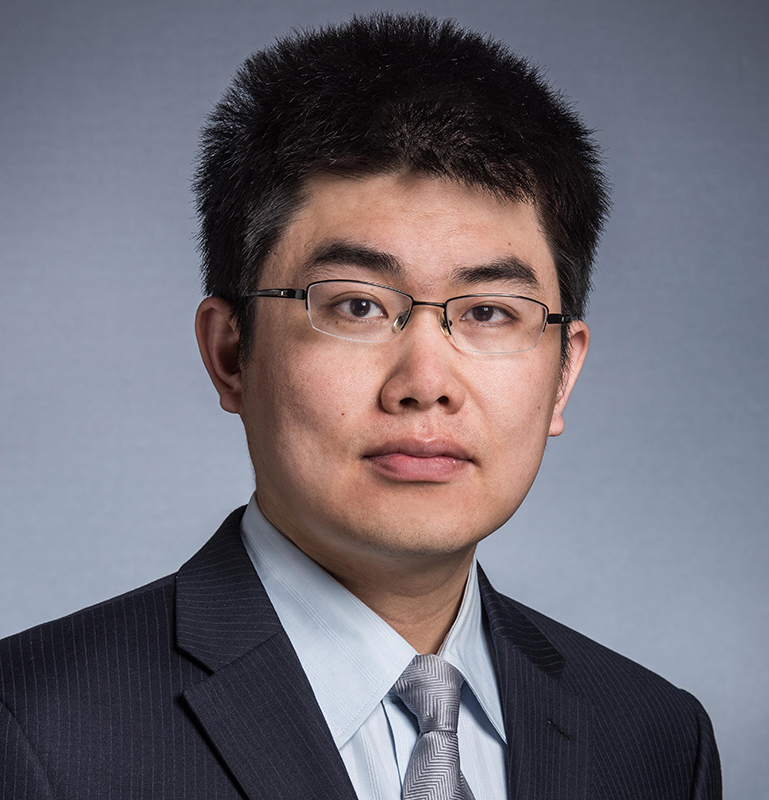The image is a close-up portrait of an Asian man, possibly in his late 20s or early 30s, dressed in business attire against a light blue-gray professional background. He has a serious, expressionless look as he stares straight ahead. His hair is black, slightly long, and fluffy, giving it a somewhat spiked and bushy appearance. He wears rectangular eyeglasses with a rimless design on the bottom and a thin gray metal frame on top and sides. His suit is dark navy blue with subtle white pinstripes, and you can see him from the shoulders up. Under the suit, he dons a light blue collared shirt paired with a light blue patterned tie with angular, L-shaped lines. The overall image suggests a formal, polished look typically used for business profiles or professional purposes.